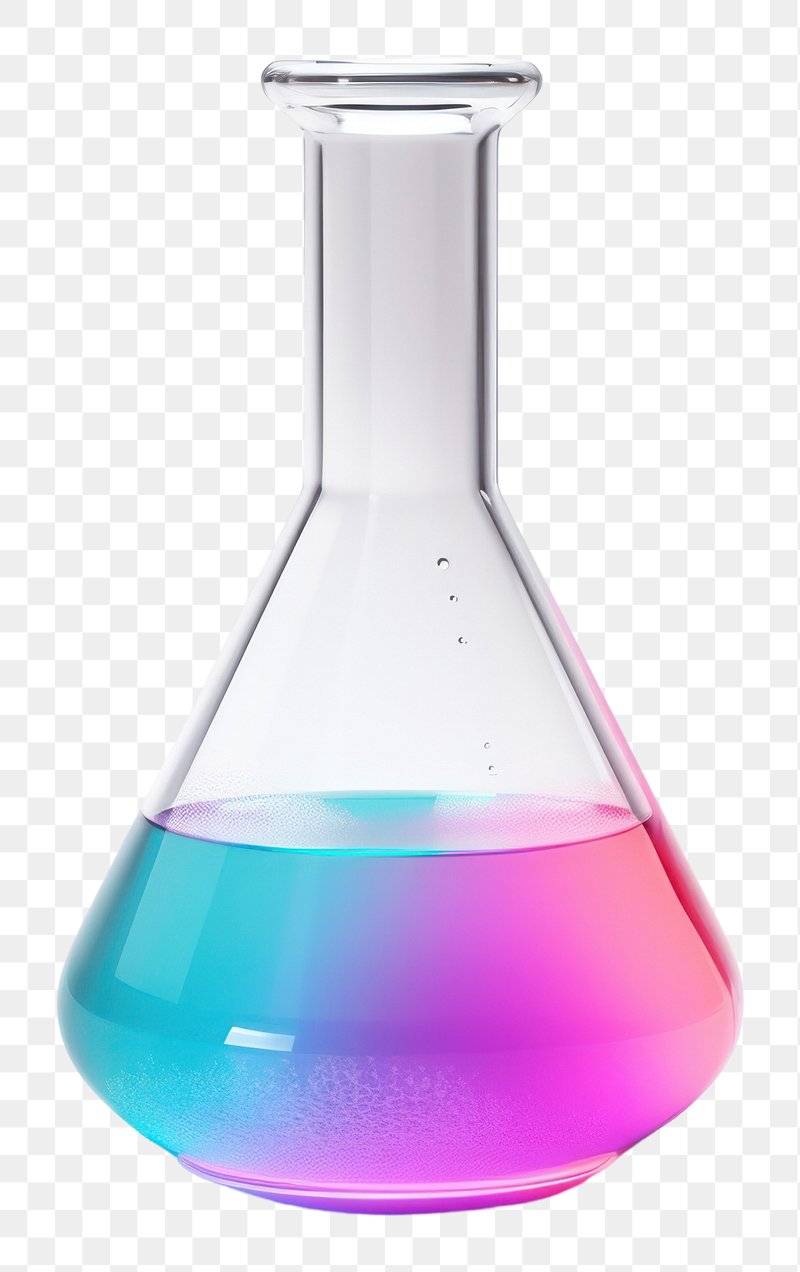The image displays a vertical rectangular graphic of a glass science flask with a narrow, rounded top that flares into a broader, triangular-shaped body. The flask is filled halfway with a liquid that exhibits a gradient of vibrant colors: deep blue on the left side, transitioning to purple in the middle, and culminating in a red hue on the right side. The background is a white and gray checker pattern, contributing to the flask's slightly opaque appearance that obscures any view through it. A subtle white reflection can be observed on the left side of the flask, adding to its glassy realism. The liquid's surface inside the flask shows a prominent purplish streak where the colors blend. The overall style of the graphic suggests it might be created within a digital art or design software.